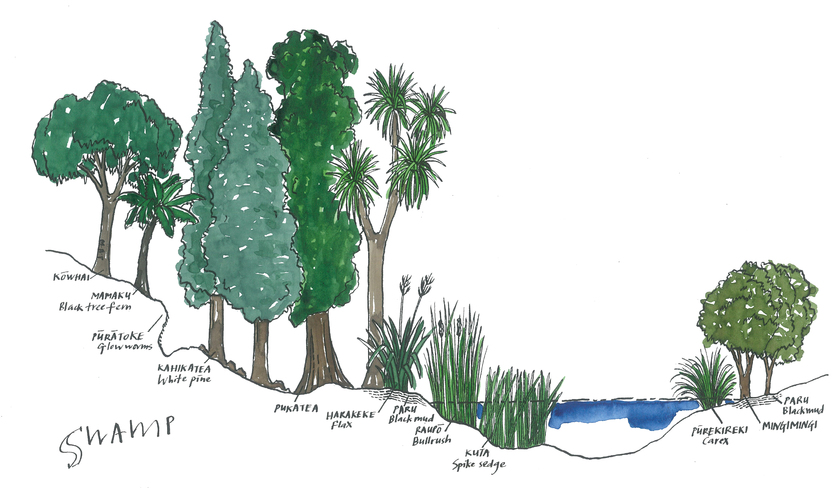The image is a detailed diagram on a white background, illustrating the components of a swamp ecosystem. At the bottom, the word "swamp" is prominently written in black. The diagram visually progresses from left to right, showing a gradient descending from higher to lower elevations into the water, then slightly back up. It features a variety of trees and plants, each identified by name. Starting from the left are trees labeled as "Kowhai," "Black Tree Fern," with a note on "Mamaku" as its alternate name, and "White Pine," also known as "Kahikatea." The sequence continues with "Pukatea," and then transitions into different types of flora such as "Harakeke Flax," "Palm Black Mud," "Bulrush," "Spike Sedge," "Kara," and "Mingi Mingi." The trees have brown trunks and green leaves, and the different plant species include tall leaves and bushy structures. The illustration, likely hand-drawn with markers or watercolor, provides a comprehensive visual representation of swamp vegetation, mentioning unique and tropical-sounding names that might be associated with a Hawaiian context.